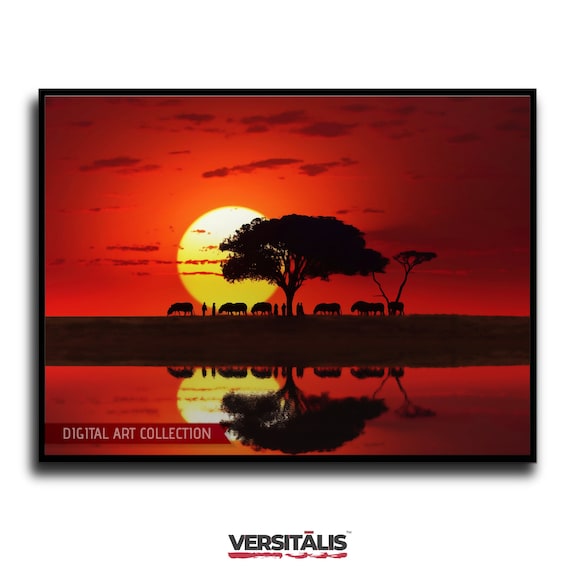The image depicts an African-inspired landscape bathed in varying shades of red, transitioning from deep red on the right to brighter red towards the left. At the center of this striking scene stands a large acacia tree, flanked by a variety of animals and people, all rendered in silhouette. The sun, positioned slightly left of center, casts a warm, yellow-orange glow, creating a dramatic backdrop along with scattered high cumulus clouds. These clouds, outlined in grayish-blue, add depth to the skyscape. Beneath the horizon, a brown rectangle spans the width of the image, reflecting the entire scene above in a serene body of water, reminiscent of a wide river or lake. In the lower left corner, a red rectangle with the inscription "Digital Art Collection" in white indicates the piece’s title or series. The overall composition, with its mirrored reflections and rich color gradients, evokes the tranquil beauty of an African sunset.